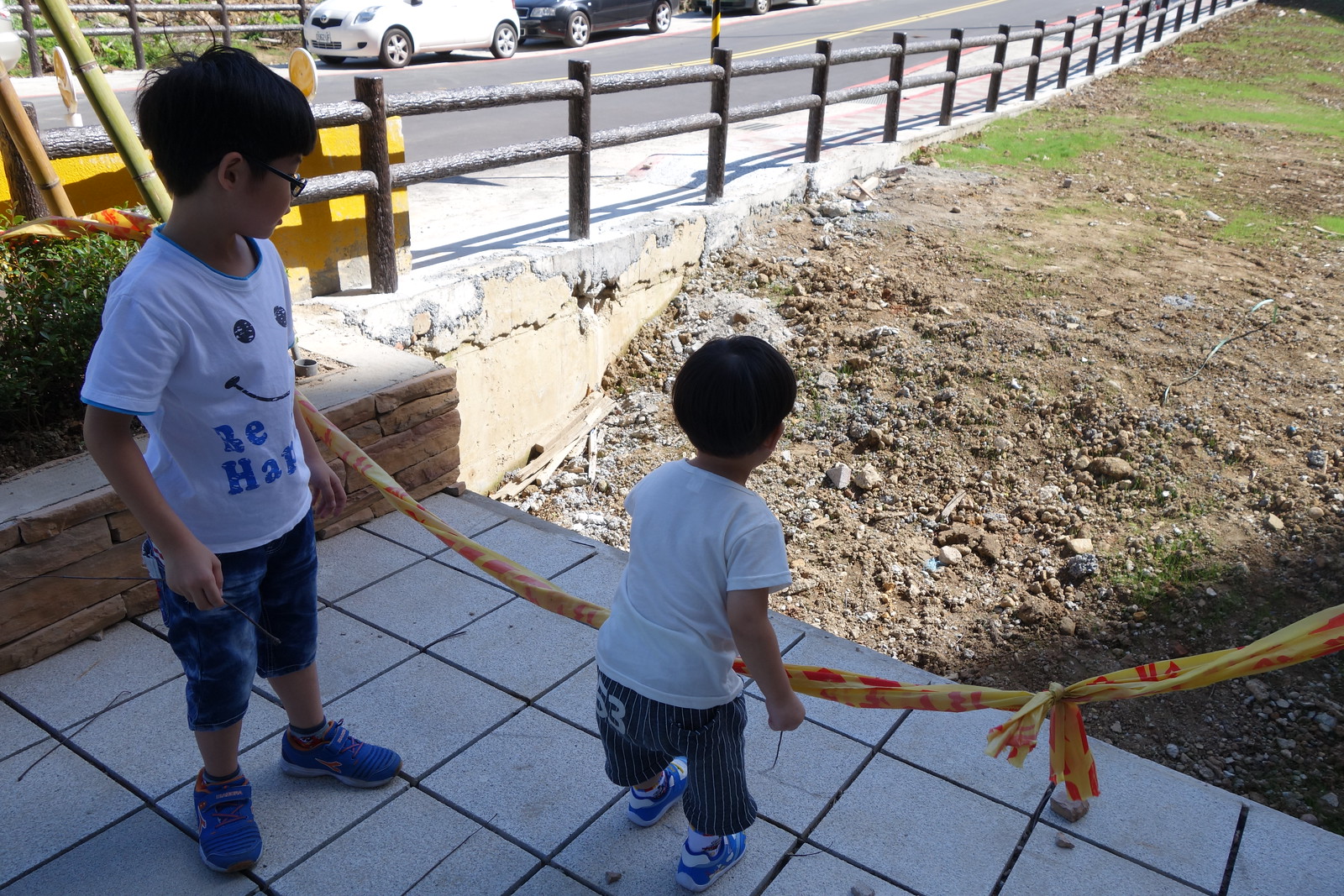The photograph captures a scene of two young children standing on a tiled deck that overlooks a construction area with a dug-up ditch. The deck, lined with large white tiles, features a low stone wall with a small plant. A yellow rope with red writing stretches across the deck to prevent access to the ditch below, which is filled with dirt and bordered by some grass. Both children, who appear to be of Asian descent, have short dark hair and are dressed in white t-shirts, shorts, and blue tennis shoes. The younger child, around three years old, attempts to touch the rope, while the older one, possibly five or six and wearing glasses, stands beside him. Beyond the ditch, patches of grass extend to a wooden post fence running alongside a two-lane road where several cars are parked.